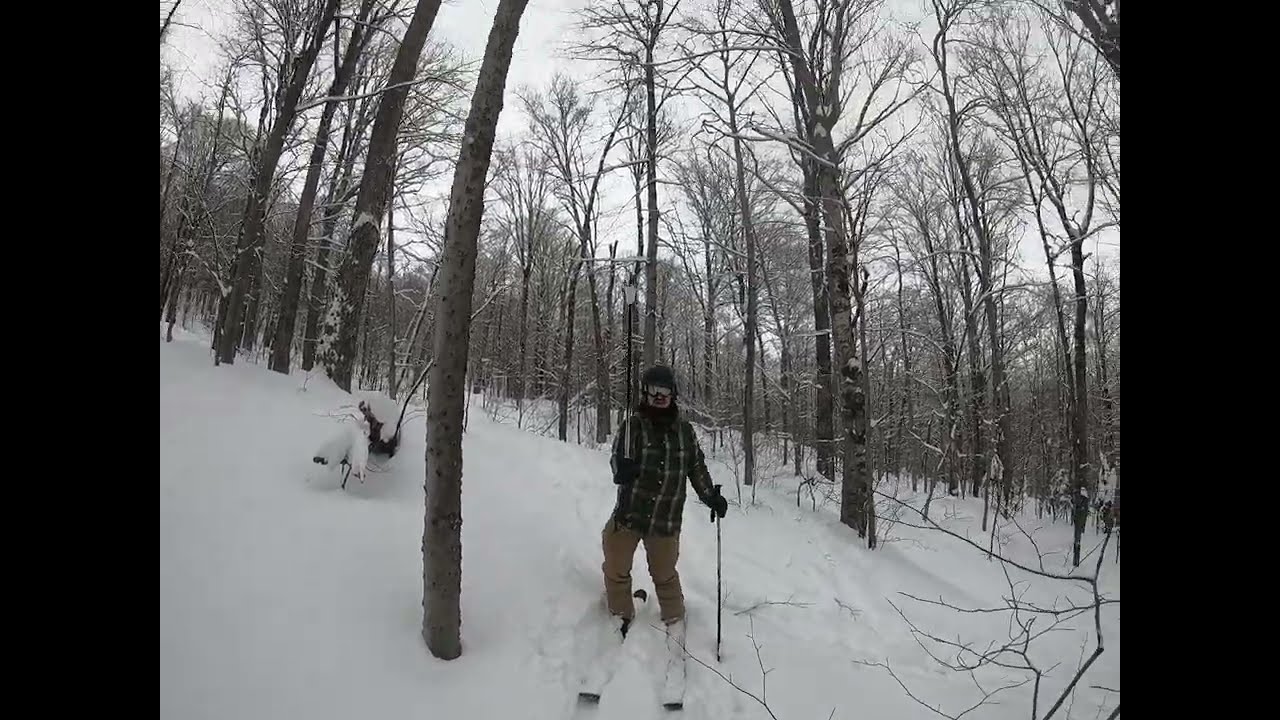In this detailed photograph taken in a hazy, cloudy daytime during winter, a solitary skier is positioned in the midst of a densely forested area. The scene is bordered by vertical, narrow black rectangles on each side, with the central image forming a large square. The sky is bright and overcast, casting a diffused light over the landscape. The ground is blanketed with thick, white snow, and the numerous tree trunks are thin and devoid of leaves, with some branches lightly dusted with snow.

The skier, whose gender is indistinguishable, is dressed in brown pants, a plaid button-down shirt or coat, and a black hat. They also wear a ski mask and goggles, obscuring their facial features, but a hint of a brown mustache can be seen. In their left hand, they hold a ski pole, while something indeterminate is held in their right hand. Their skis are strapped to their feet, though partially covered with snow, suggesting recent movement. The skier stands, gazing directly at the camera, giving the impression of a selfie in a tranquil yet expansive, wooded snowscape. The image conveys a sense of solitude and the skier's search for an open space to continue their skiing adventure amidst the crowded trees. There are no other people or animals in sight, emphasizing the skier's solitary journey.